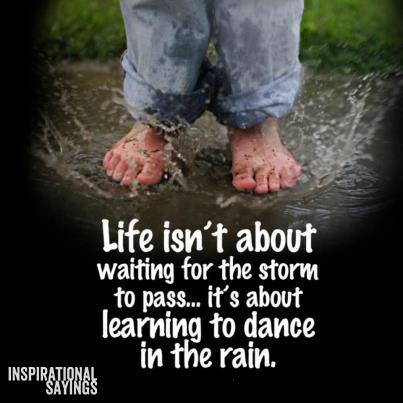The image is an advertisement featuring a motivational message. The top section of the image captures a photograph showing a pair of bare feet splashing in a puddle, seemingly just landed, sending water droplets around. The person is wearing light blue jeans with cuffs rolled up, now soaked from the puddle. The ground beneath appears to be a gray concrete sidewalk, with a small patch of grass visible in the background. The individual has fair skin. The entire scene is set against a stark black backdrop, which contrasts sharply with the vibrant elements in the photo.

Below the image, in white font, is an inspirational quote: "Life isn't about waiting for the storm to pass; it's about learning to dance in the rain." In the bottom-left corner, the words "inspirational sayings" are also displayed. This image, with its blend of vivid colors and empowering text, resembles a motivational poster or a graphic that might be shared on social media.